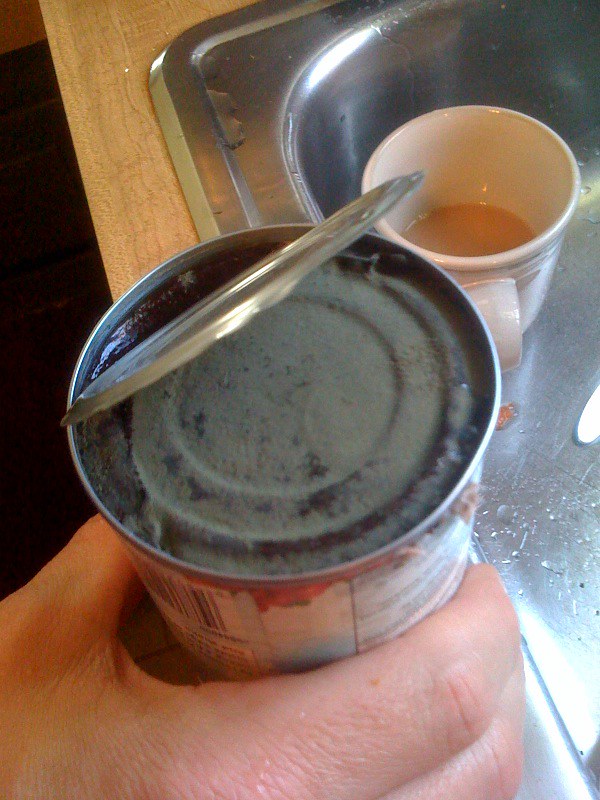This detailed photograph, taken indoors in portrait mode, captures a close-up of a Caucasian man's right hand holding an upside-down, open can at the edge of a stainless steel kitchen sink. The lid of the can is still attached, revealing a grayish, black material inside that appears unappetizing, possibly spoiled, with concentric rings, suggesting it could be a bean paste or another food item that has gone moldy. A white and red label partially wraps around the can, displaying part of a barcode. In the sink sits a white ceramic coffee cup containing a small amount of light brown liquid, likely coffee with cream. The surrounding counter is wood-toned.